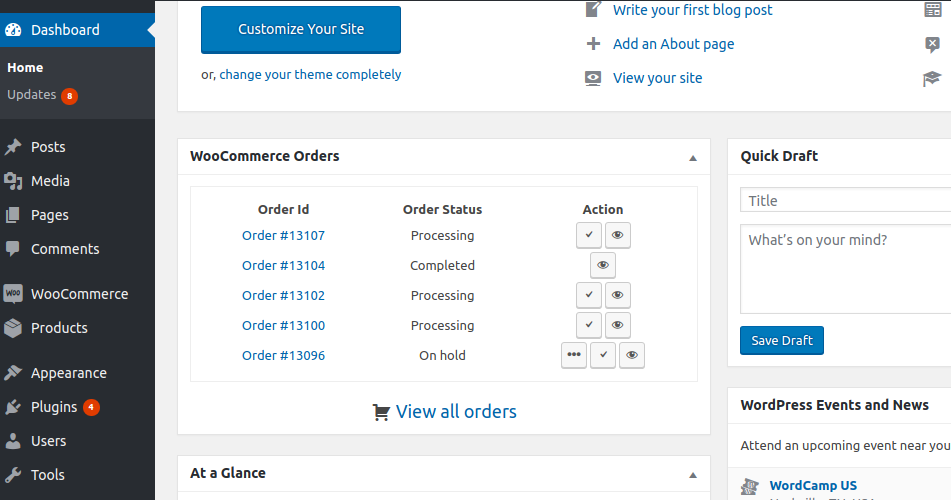This image showcases a detailed view of a computer dashboard associated with a content management system. On the left side, a vertical black sidebar features a prominent blue banner at the top labeled "Dashboard." Below, it enumerates various categories: "Home," "Updates" (adorned with a red circle displaying the number 8), "Posts," "Media," "Pages," "Comments," "WooCommerce," "Products," "Appearance," "Plugins" (accompanied by another red box indicating 4 updates), "Users," and "Tools," each paired with corresponding icons.

The main area at the top highlights a call-to-action section encouraging users to "Customize Your Site" with a blue button or "Change Your Theme Completely." Below this, a prominent white box labeled "WooCommerce Orders" lists the details of five distinct orders, including their order ID numbers (in blue) and their respective statuses like "Processing," "Completed," or "On Hold." A "View All Orders" link at the bottom, symbolized by a shopping cart icon, provides additional navigation options.

Additionally, the top of the main section prompts users to "Write Your First Blog Post," "Add an About Page," or "View Your Sites," each suggestion accompanied by relevant icons. To the right, there is a compact "Quick Draft" box for users to jot down their thoughts, featuring fields for "Title," "What's on Your Mind," and a blue "Save Draft" button.